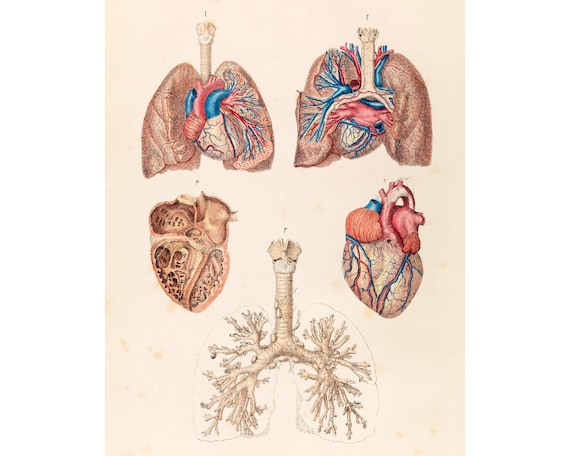This anatomical illustration, set against a vivid pink page, features detailed images of the human heart and lungs, likely excerpted from a medical reference book. The top left illustration showcases a pair of pink lungs connected to a descending trachea. Adjacent to it, a detailed depiction of the heart highlights the complex network of red arteries and blue veins emerging from it. The next illustration on the right provides a cross-sectional view of the lungs, emphasizing the intricate network of veins and arteries in contrasting blue and red hues, along with a prominent red artery traversing the lungs. Below the initial set of lungs, we observe a halved heart, rendered in pink, revealing its internal chambers and structure. To the right of this, another heart illustration focuses on the detailed vasculature on its exterior, rich in color and intricate detail. The bottom image culminates with an in-depth view of the interior lung anatomy, further highlighting the meticulous structural intricacies within.